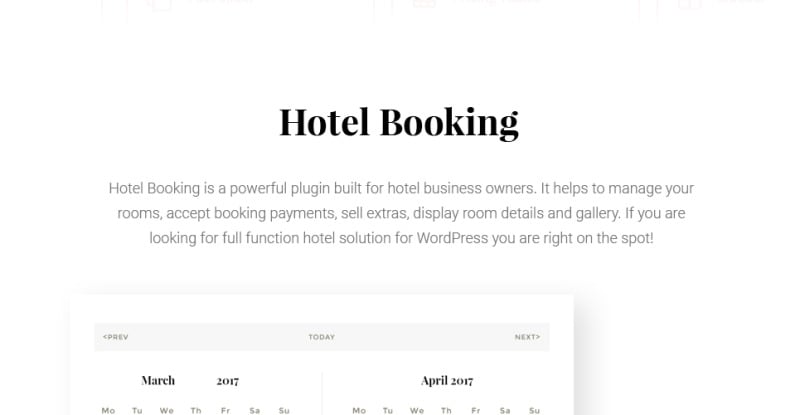Partial view of a website home page showing a powerful hotel booking plugin. The prominent title "Hotel Booking" is displayed in bold black font. The plugin is designed specifically for hotel business owners, enabling them to manage rooms, process booking payments, sell additional services, and showcase room details in an image gallery. The descriptive text is center-aligned and presented in a light gray color. Below this, there is a calendar section within its own box. The top navigation includes "Previous" with a left arrow, "Today" centered, and "Next" with a right arrow. The calendar displays the months "March 2017" and "April 2017" along with the days of the week listed underneath.